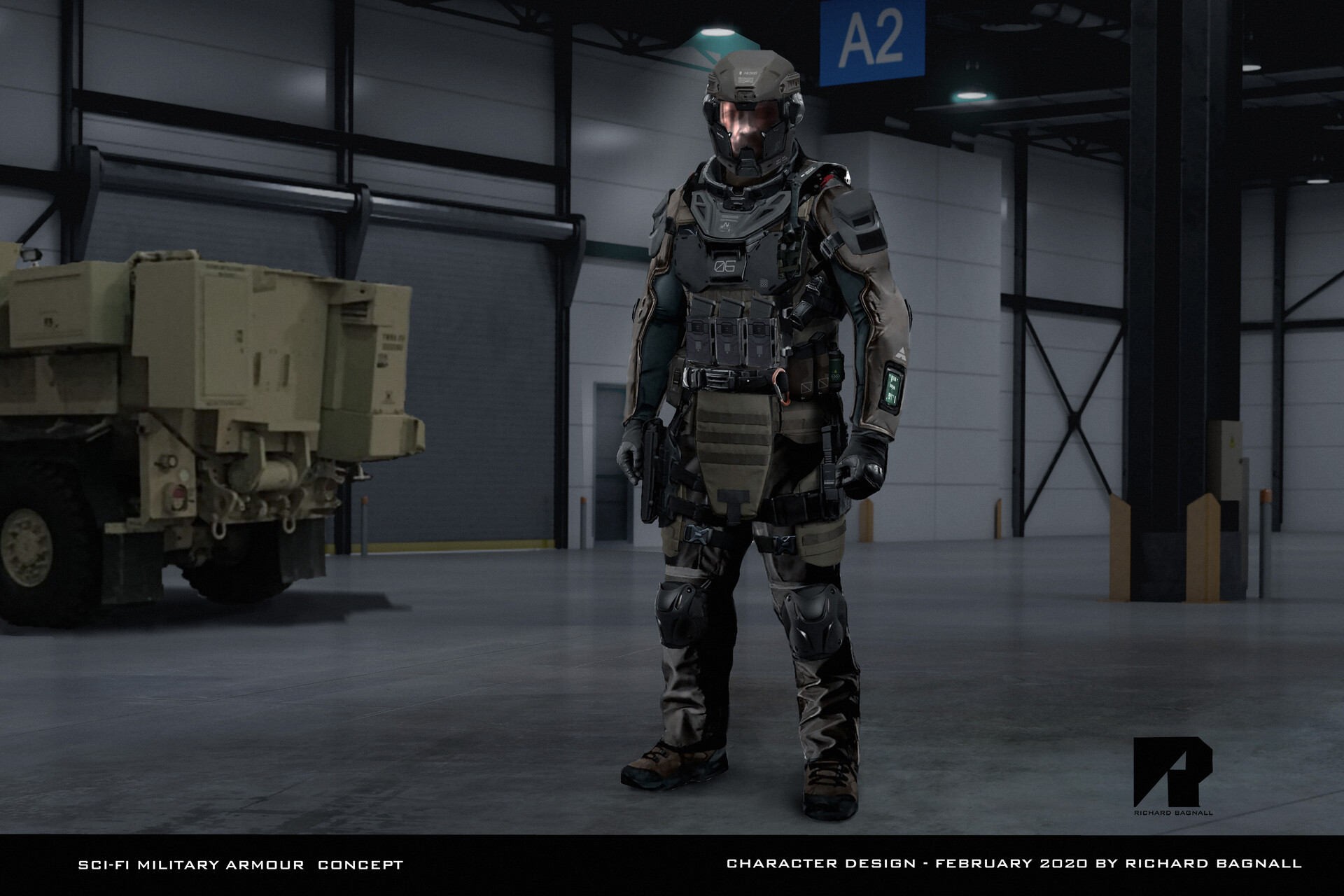The image showcases a 3D concept design of a science fiction soldier situated in the center of a warehouse. The soldier, adorned in advanced, futuristic armor, stands prominently against the backdrop of a tall white wall on the back of the warehouse. The wall features a large rolling garage door alongside a smaller gray push door. On the right side, a tall black support beam is encircled by yellow protective bollards, ensuring its safety from impacts. To the left, the rear of a tan-colored military truck is visible. At the bottom of the image, a black banner spans from right to left, displaying white text that reads: "sci-fi military armor concept character design February 2020 by Richard Bagnall." The color palette in the scene includes shades of gray, green, black, white, blue, pale yellow, and beige. The design is highly detailed and appears to be a still from a game trailer, with the logo of the game company positioned in the bottom right corner.